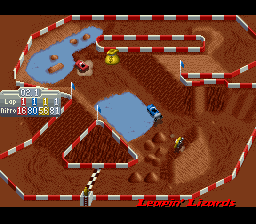The screenshot depicts a vibrant and whimsical race track from a video game, characterized by its playful design and colorful elements. The race track, outlined by a prominent red and white barrier, guides the racers through its course, ensuring they stay on track. Strategically placed along the barrier are white poles supporting blue rectangular flags, signaling specific points of interest or caution.

Prominently displayed in the lower right-hand corner of the screen is the playful text "Leapin' Lizards," emphasizing the game's lighthearted nature. On the left-hand side, the display indicates the player is on lap 1. Below this, a "Nitro" meter showcases the player's nitro levels with precise measurements: 16 (red), 80 (blue), 56 (yellow), and 81 (white). Above this meter, a small grid or key is labeled "02.1."

The scene features three cars: a blue car positioned near a small water hazard, a red car confronting a larger water hazard with embedded rocks, and a tipped-over yellow car right at the track's beginning. These cars add to the dynamic and engaging visual experience, indicating that this could be a child's game with its simple yet captivating graphics and elements.